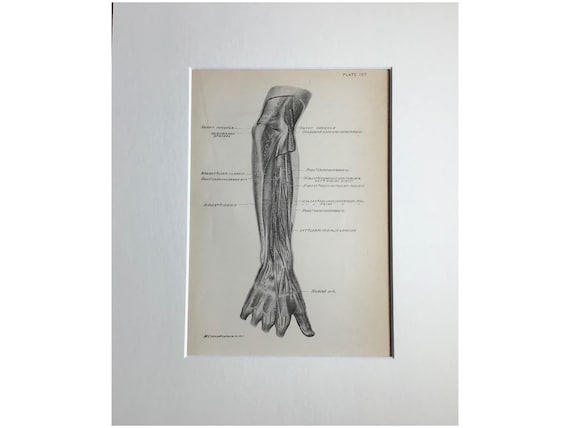The image is a detailed black and white illustration of a human arm, from just above the elbow to the second joint of the fingers, depicted on an old, worn, yellowed page that resembles a matted photograph from a medical textbook. The illustration appears to be hand-drawn, likely in graphite pencil or pen and ink, showcasing the internal structures such as muscles, veins, and bones, including the hand and fingers. These anatomical features are meticulously labeled with lines pointing to various parts, although the text is too small and blurry to be legible. The arm is shown in a cutaway view, probably intended for educational use, possibly in a medical school context. The background is a vanilla color, enhancing the contrast of the black and white shading, which brings out the intricate details of the musculature, vasculature, and skeletal elements. Despite the blurriness of the labels, the depicted arm serves as a fascinating instructional or demonstrative tool.